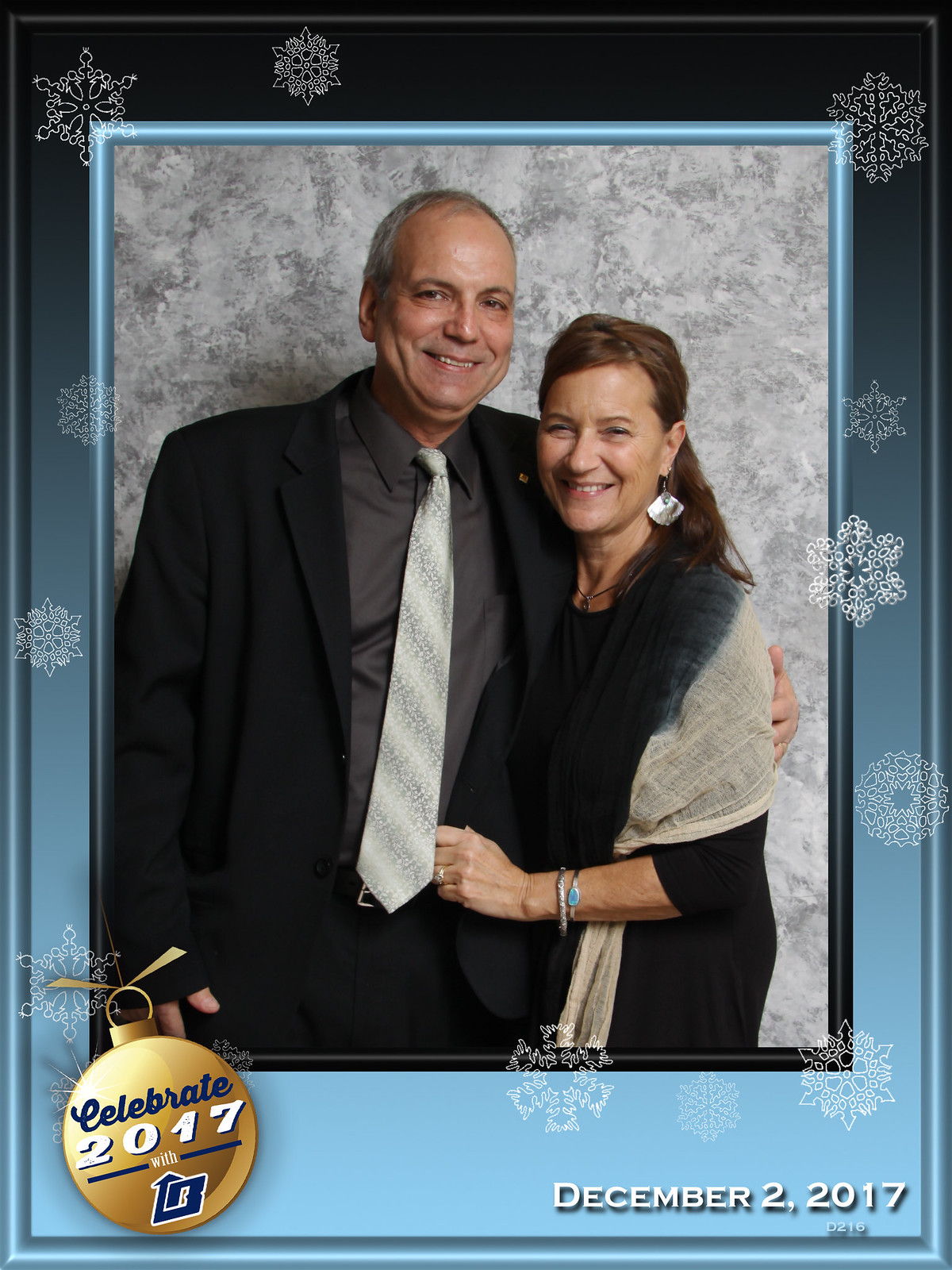In this intricately detailed picture, we see an image of an elderly couple captured within a central photo frame, which features blue borders. This smaller frame is set inside a larger frame with alternating blue and blackish borders. The background surrounding these frames boasts elegant white floral and designer patterns. 

In the bottom-left corner of the outer frame, there is a distinctive logo resembling a golden ball with a ring on top, accompanied by the text "Celebrate 2017" and a bee logo with an upward-pointing blue arrow. The bottom-right corner displays the date "December 2, 2017" along with the number "D216."

At the heart of the image, the old couple is smiling directly at the camera. The man, who is taller than the woman, is dressed in a black coat, black pants, a dark grey shirt, and a silver tie. He has a clean-shaven face and a balding head. The woman is wearing a black dress with a stole draped over her shoulders, along with bangles or bracelets on her left hand. She clutches the man at his stomach, showcasing a ring on her ring finger and silver earrings that match her brown hair. The backdrop for the couple is a wall adorned with a greyish patterned wallpaper.